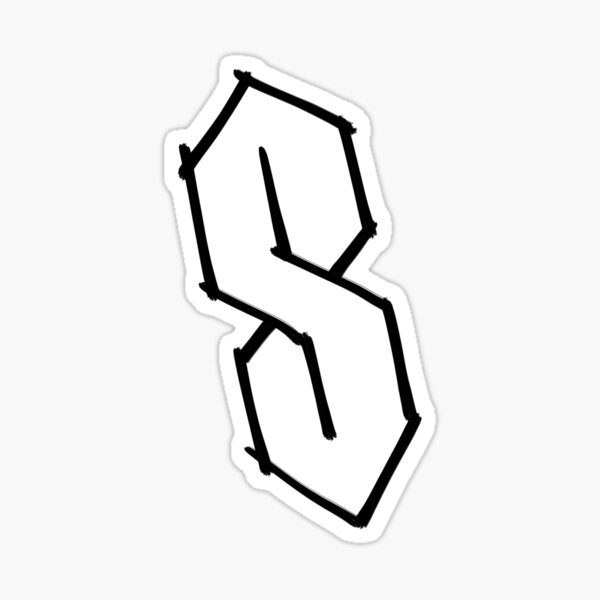This image depicts a detailed drawing resembling a "cool S" or "Super S" sticker, popular in the 80s and 90s, known for its stylized, intricate, and somewhat 3D appearance. It features a prominent, thick black outline contrasted against a stark white interior. The backdrop is a plain white surface. The S's design is characterized by its composition of straight lines and diagonals, avoiding any curves. The lines extend slightly beyond their intersection points, giving it a layered and dynamic look. The S starts with a central vertical line, followed by alternating diagonal and straight lines to create a continuous, interconnected pattern. The entire S appears slightly tilted to the left, occupying the center of the image, with no additional text or context surrounding it.